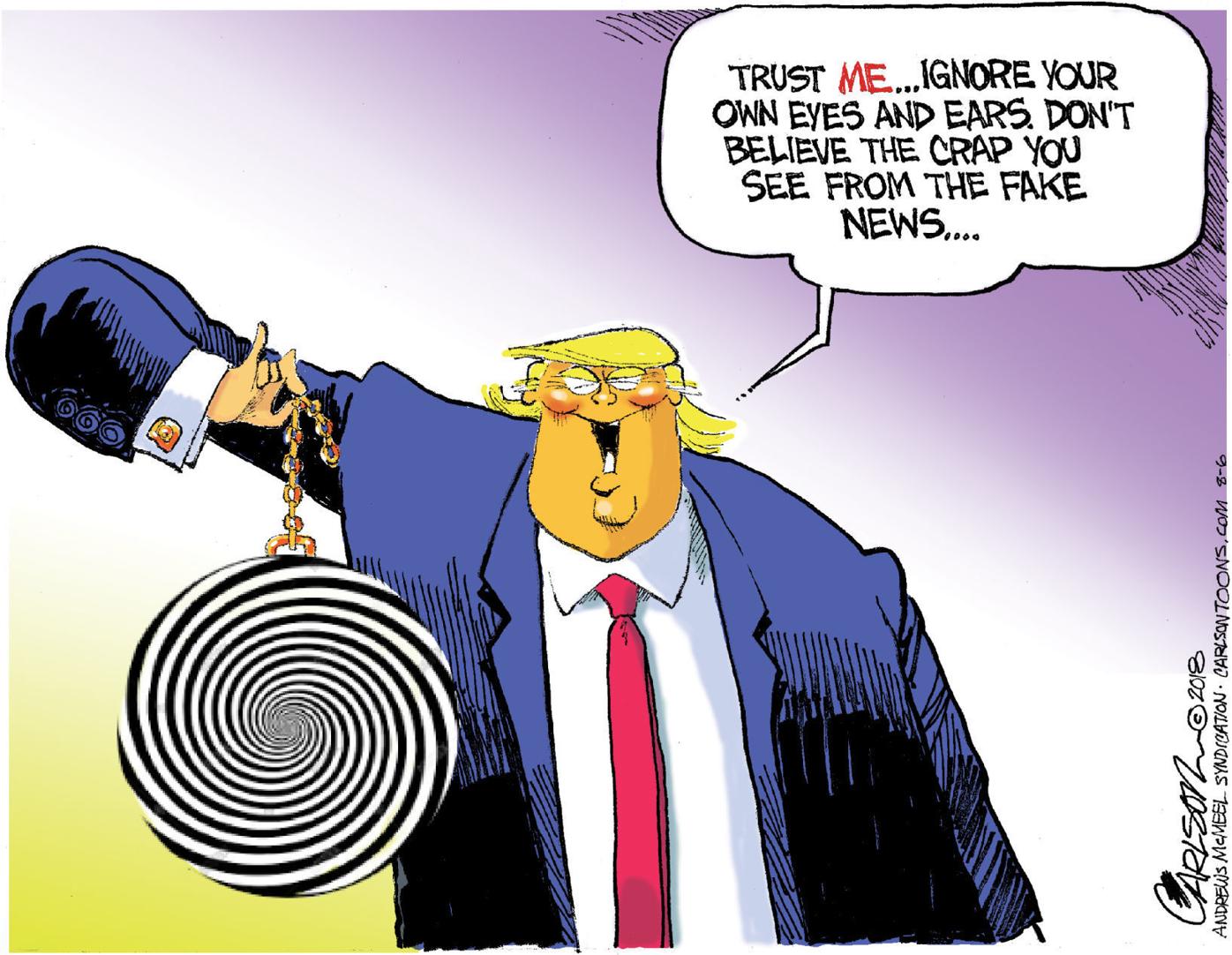In this political cartoon, a caricature of Donald Trump, the former U.S. President, is front and center, facing the viewer with an exaggerated version of his distinctive features—his yellow hair, blue suit, white collared shirt, and red tie. The cartoonist has taken creative liberties to accentuate his appearance, portraying Trump from a low angle, giving the impression that he is looking down at the viewer. In his right hand, he dangles a large, comical hypnotic device, resembling a pocket watch with a swirling pattern meant to suggest hypnosis. In the top right corner, a speech bubble reads, "Trust me... ignore your own eyes and ears. Don't believe the crap you see from fake news." This ironic setup lampoons Trump’s relationship with the media and his frequent accusations of "fake news." Along the side of the image is the signature reading "Andrelis McMeal syndication," identifying the cartoon's creator and its intention to be humorous and entertaining.